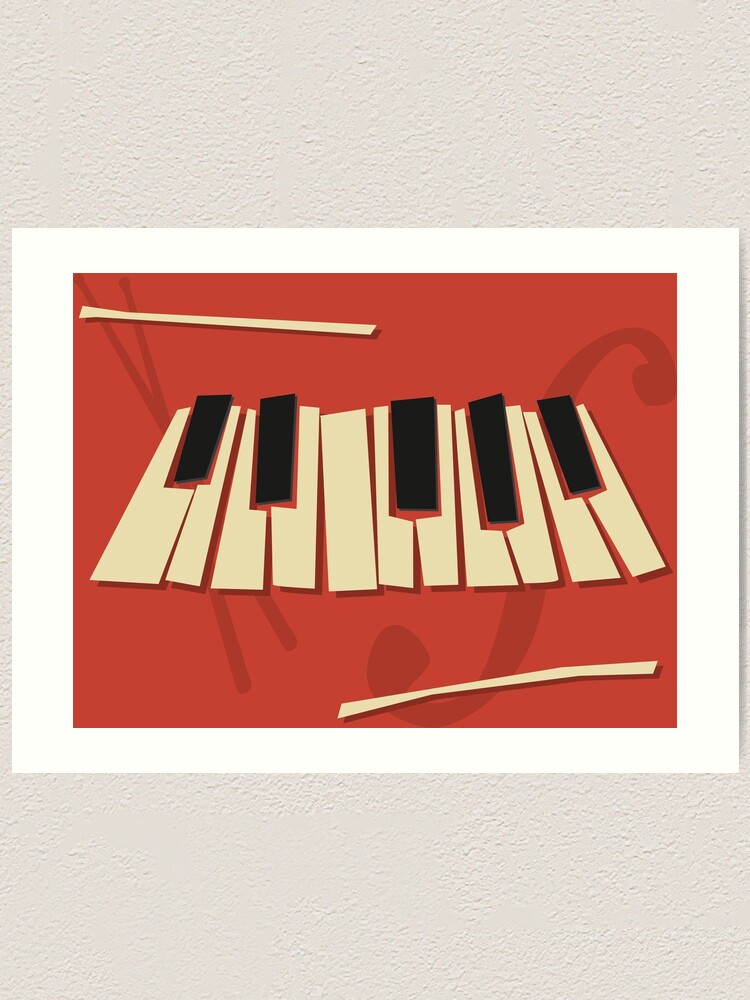This photograph captures a framed artwork mounted on a white wall. The artwork features a highly stylized and somewhat impressionistic depiction of piano keys, rendered in clean, digital lines. Unlike a traditional keyboard, the keys in this digital drawing are irregular polygons that create an uneven, asymmetrical pattern. The instrument, resembling a Zamboni or perhaps a xylophone, is composed of a series of keys with unique spacing: five black keys outlined in red, each flanked by two long, rectangular white keys that are split to fit around the black ones. Notably, one white key stands alone without a corresponding black key. The arrangement follows a sequence of alternating keys: white key, black key (centered), white key, white key, black key, and so forth. Also depicted are two thin, white sticks—one positioned beneath the row of keys and one across the top. The background of the artwork is a vibrant red, adorned with dark red curlicues, providing a striking contrast to the beige and black keys. The image is set within a cream-colored frame, adding an additional layer of depth to the composition.